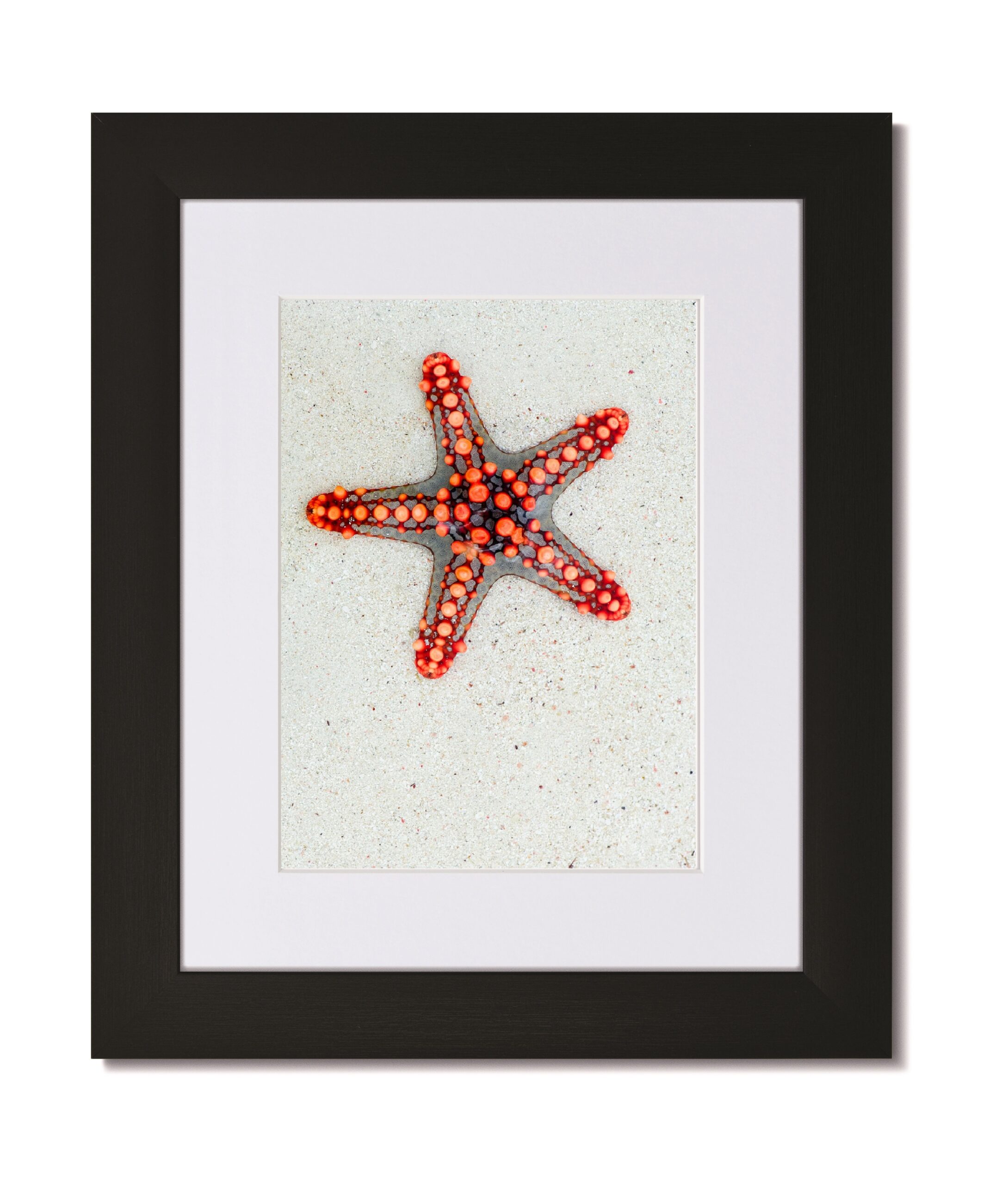The image depicts a meticulously framed artwork featuring a man-made starfish, likely crafted for an art project. Enclosed in a bold, thick black rectangular frame, the artwork is accentuated by a white beveled mat that proportionally follows the frame’s lines. At the heart of the composition is the starfish, rendered in a delicate, almost translucent gray material. Its five arms are adorned with pearly pinkish-orange bubbles or beads that graduate in size, with the smallest beads near the arm tips and enlarging towards the center. Positioned on a backdrop that resembles fine white gravel sand or a tan marble surface, the starfish's arms convey a sense of meticulous, deliberate craftsmanship, enhancing the striking visual contrast against the light background.